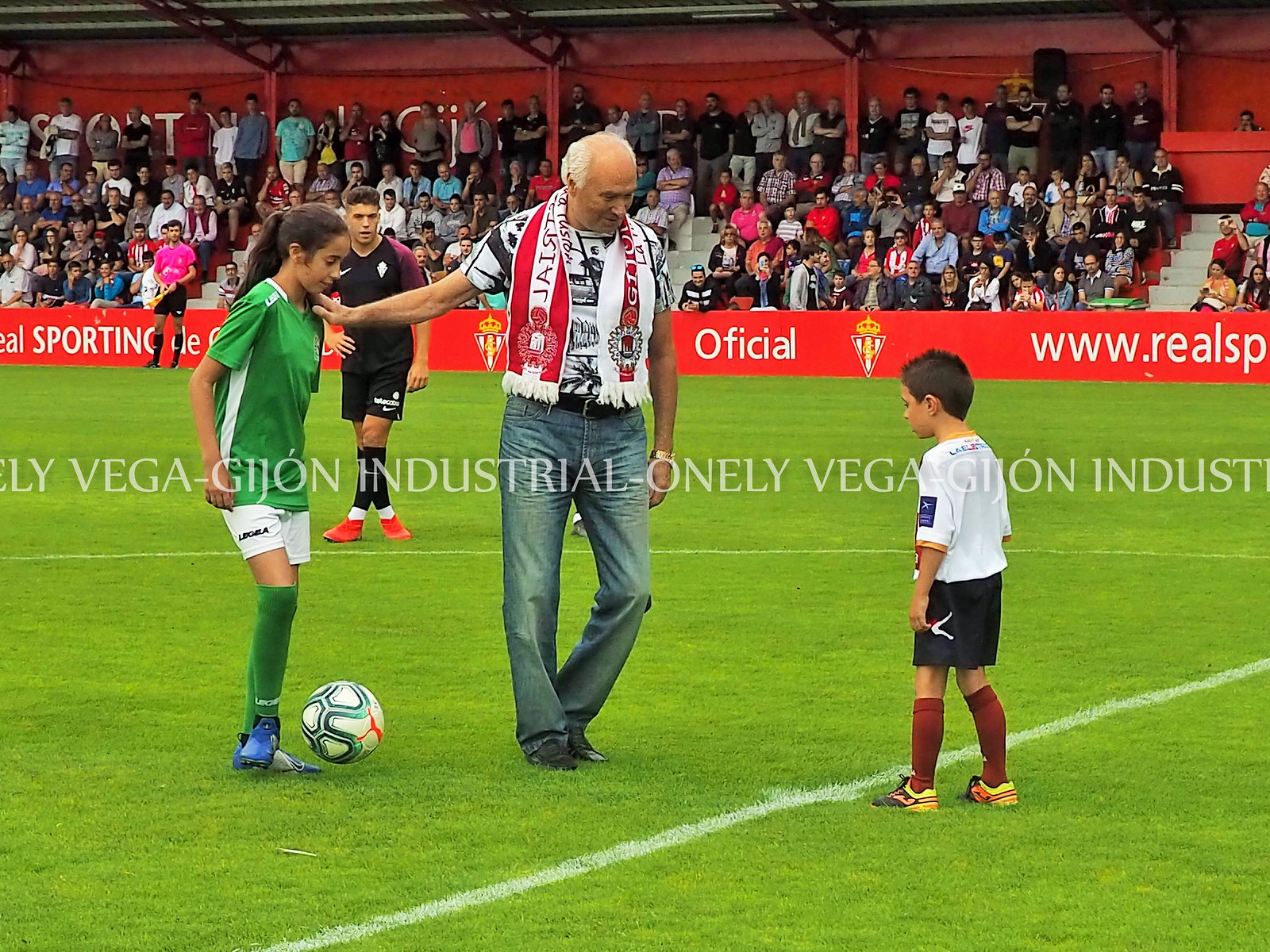In this photo taken at an outdoor soccer stadium, a green grass field is the main focus, bordered by a red barrier in the distance. The stands are filled with numerous spectators sheltered under a canopy, creating a lively atmosphere. Prominently in the middle of the field stands a man dressed in blue jeans and a black and white shirt, with a scarf around his head. He has his hand on the shoulder of a young girl who appears to be around 9 or 10 years old. The girl, with long brown hair tied back in a ponytail, is dressed in a green soccer jersey, white shorts, green socks, and blue shoes. In front of her is a soccer ball that’s white, green, and red. Across from her stands a much younger and shorter boy, perhaps half her age. He is dressed in a white jersey, black shorts, and crimson red socks, with short brown hair. They seem poised for a playful moment of soccer interaction. In the background, towards the side of the field, another soccer player dressed in black and red can be seen, as well as a boy in a black shirt and shorts.